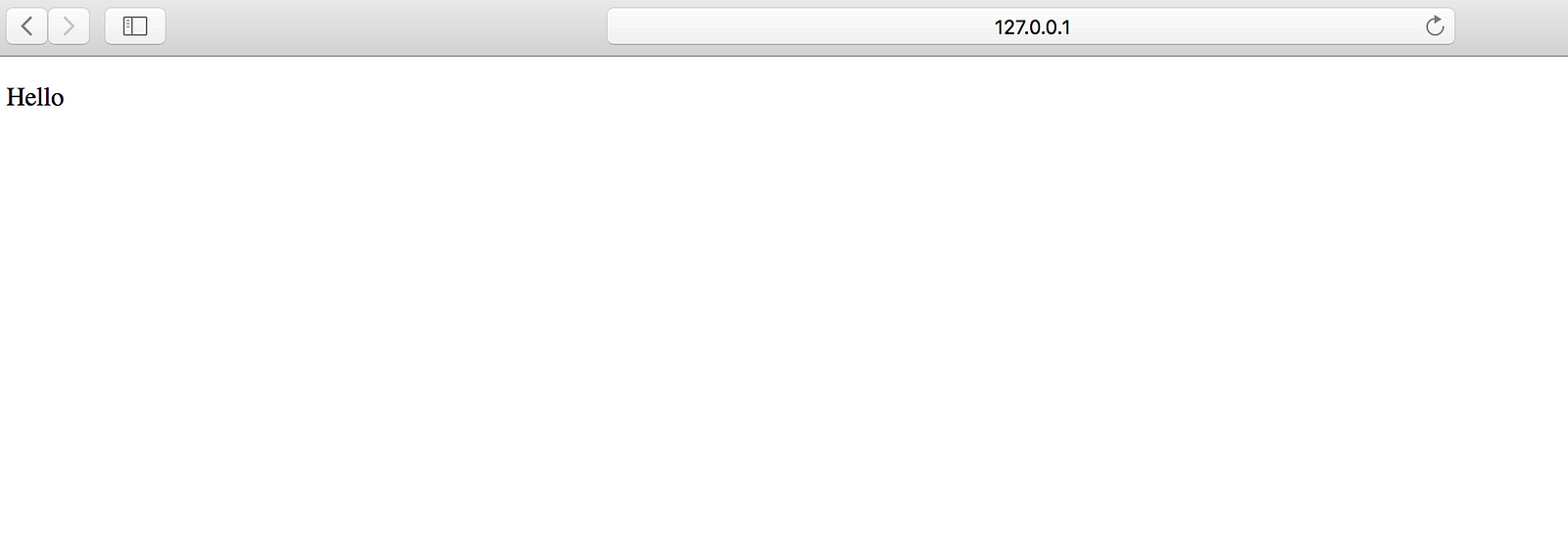Here we have an image depicting a web browser window, likely displayed on an Apple or Mac device. The top of the browser showcases a light gray or silver-colored title bar. On the upper-left side of this bar, there are three square icons. The first square has a light gray background and features an arrow pointing to the right. Directly to the right of this, there's another arrow symbol, this time in a lighter, almost faded gray, also set against a light gray background. Further right, there's an icon resembling a book or page, enclosed within a light gray square. On the far right of the title bar, a white address bar displays the numbers "127.0.0.1", with a refresh symbol situated at the far right end of this bar. Below the address bar, black text in bold letters reads "hello".